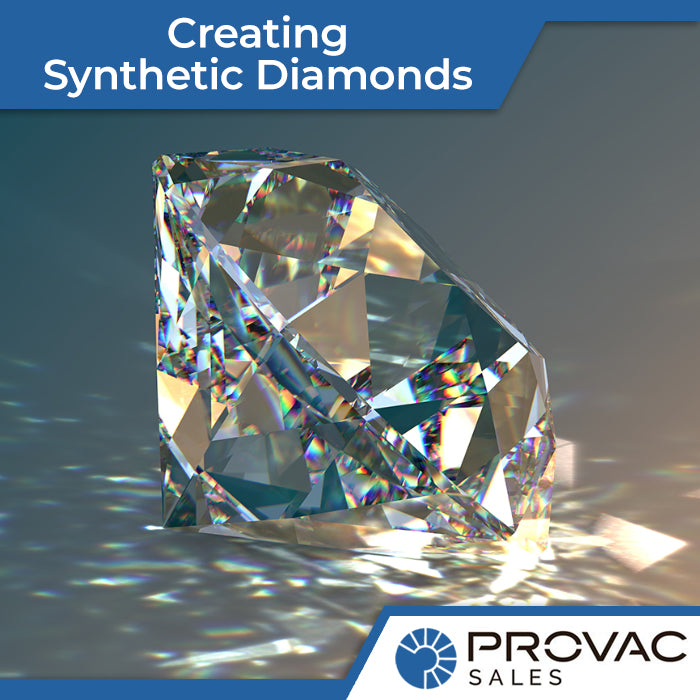The image features a clear and detailed photograph of a beautifully cut diamond, likely an American cut, resting on a darker, gray surface. The diamond, which is synthetic, is enlarged and magnified to showcase its intricate facets and brilliant reflections. Light, either sunlight or another source, penetrates the diamond, creating rainbow-like reflections both within the gem and on the surface beneath it. The top of the image is bordered by a blue banner with white text that reads "Creating Synthetic Diamonds," indicating the theme of the advertisement. In the bottom right corner, the words "Provax Sales" are displayed alongside a blue and white emblem depicting a diamond-like shape with linear cut designs. The overall composition, including the light effects and the information provided, suggests this image is likely part of a sales brochure or promotional material for Provax Sales, emphasizing the high quality of their synthetic diamonds.